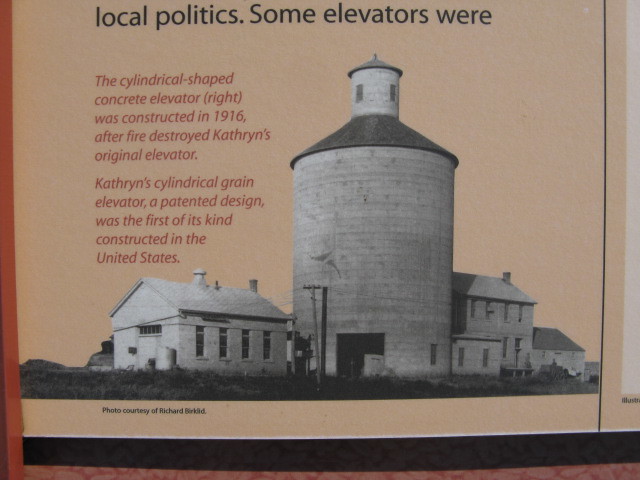This image, likely displayed in a museum, features a historical black-and-white photo of an agricultural structure, specifically a cylindrical concrete grain elevator constructed in 1916. This elevator was built to replace Catherine's original elevator, which was destroyed by fire. Notably, Catherine's cylindrical grain elevator was the first of its kind in the United States, a patented design unique for its time. The photograph includes two houses flanking the central silo, which has a smaller dome room on top with a window. The detailed write-up accompanying the image includes headers in black text stating "local politics" and "some elevators were," followed by a description in red letters detailing the history and significance of the grain elevator. The backdrop of the sign is predominantly pink, with black text at the bottom crediting the photo to Richard Birkfeld. The entire scene is depicted in a grayscale palette, emphasizing the historical nature of the photograph.